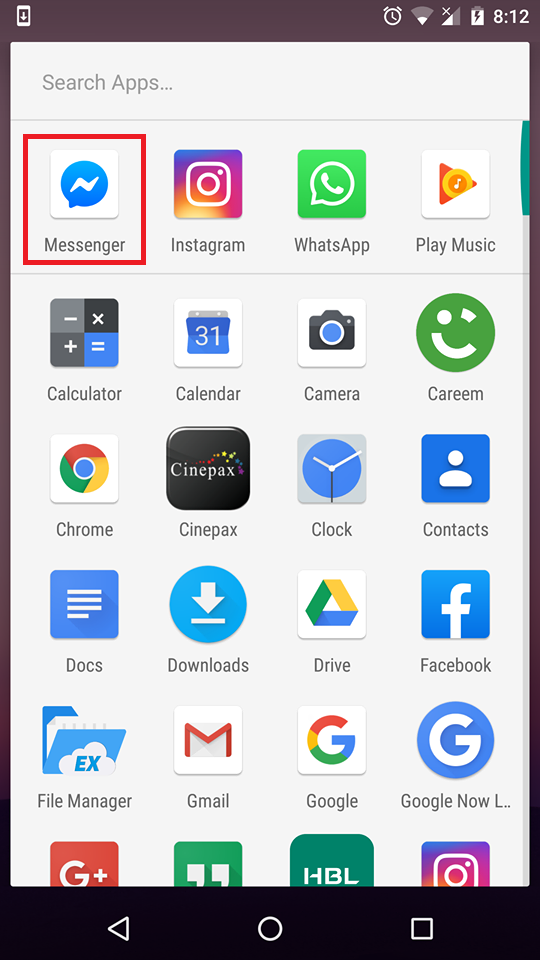In the image, the top portion is purple and features several icons. From left to right, there is a phone-like symbol with a downward arrow next to it, followed by a clock icon with arrows on its face. To its right is a WiFi symbol with an "X" at the top, indicating no connection. Next is a battery icon displaying a lightning bolt in the center, and the time shown beside it reads 8:12.

Below these icons, there is a text area labeled "Search Apps." Additionally, there is a red circle around an element with the word "White" written within it.

The image also shows various app icons. A blue bubble with a lightning bolt in the center represents Messenger. There’s an Instagram icon represented by a rounded square gradient. A green bubble labeled "WhatsApp" is present. Other app icons include Phone (in white), orange arrows (for Play Music), Calculator, Calendar, Camera, Karim, Chrome, Cinepax, Clock, Contacts, Docs, Downloads, Drive, Facebook, File Manager, Gmail, Google, Google Now, a red square, and a green square with "HPL" in the middle.

Towards the bottom is a smartphone navigation menu featuring a left arrow icon, a circle, and a square.

This detailed description provides a comprehensive overview of the icons and their layout within the image.